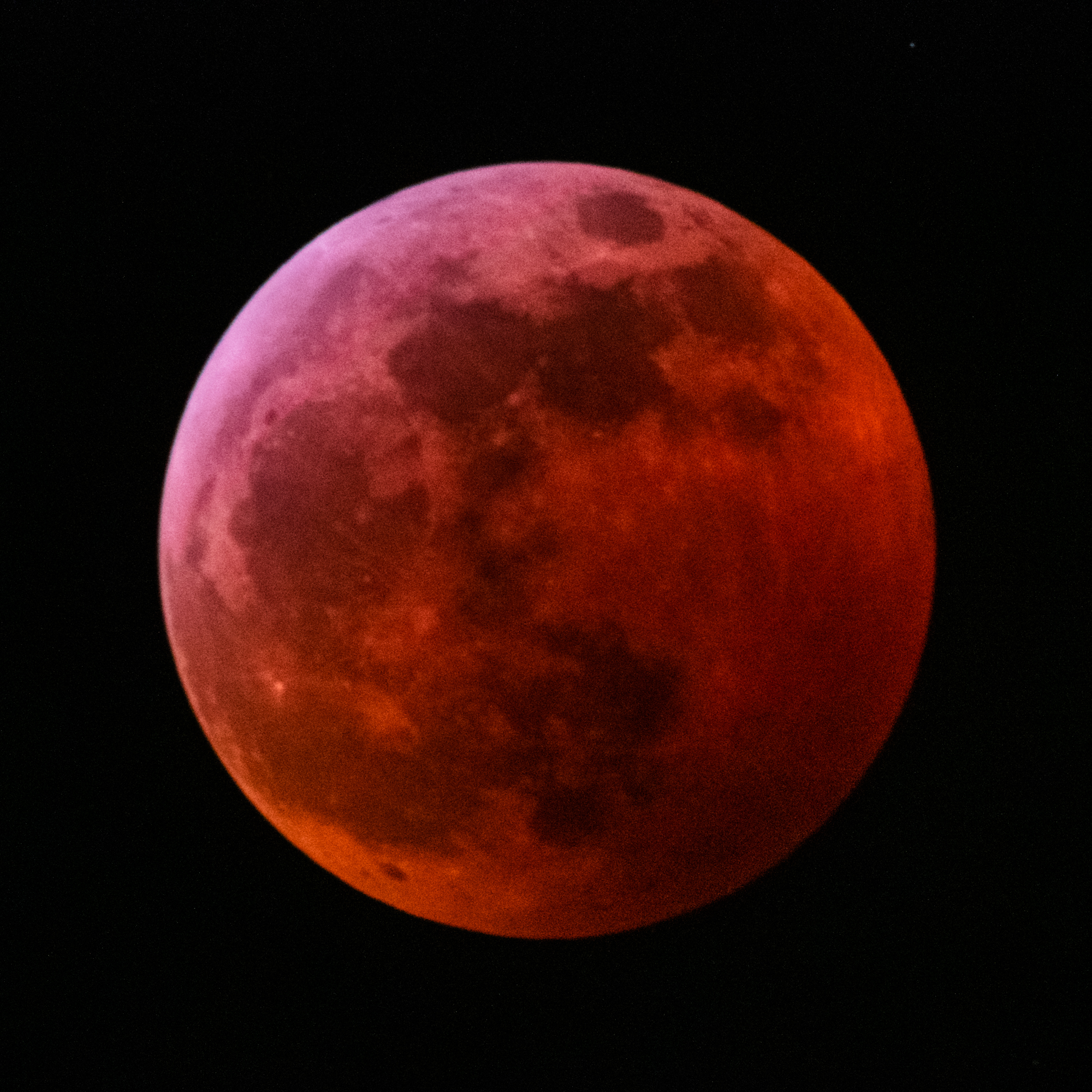The image portrays a vividly red celestial body, reminiscent of a blood-red moon or the planet Mars, suspended in a vast, empty black expanse. The focal point, this striking red orb, is perfectly circular and centrally positioned. It exhibits a spectrum of captivating hues, ranging from blood orange to dark blood red, with areas of brighter purple at the top. The surface is pockmarked with various craters and splotches, some appearing darker and others lighter, resembling round markings or ink spots. These features contribute to its rugged, rocky texture, enhancing the impression of a desolate, cratered landscape. The surrounding blackness accentuates the planet’s stark, isolated presence in space. There is no text in the image, and the overall setting conveys a hauntingly beautiful and solitary celestial scene.